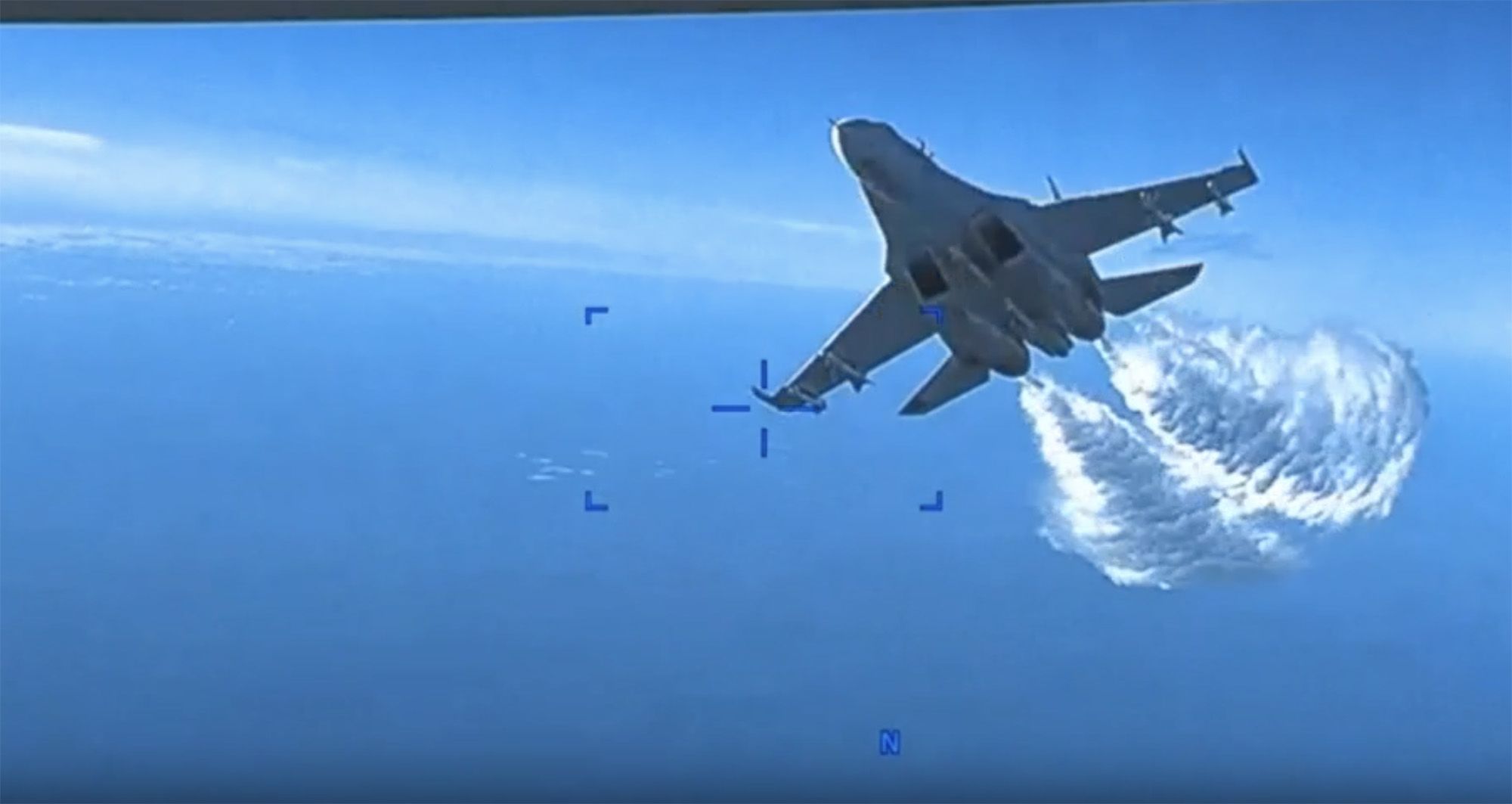The image is an outdoor color photograph taken from the viewpoint of a United States drone high in a blue, slightly overcast sky. The focal point of the image is the underbelly of a Russian fighter jet, which is positioned off-center to the left and is approaching the drone at a slight upward angle. The jet is powerful and appears to be traveling at high speed, as indicated by the two conical-shaped vapor trails of white and darker blue smoke streaming from its rear. The jet’s entirety is seen from below in shade, revealing two 'N' vents on its belly, and it carries two missiles under each wing. Superimposed over the image are crossbars and a partial blue dotted viewfinder consistent with a target acquisition system. Cirrus clouds in the deep blue sky provide a soft-focus backdrop, suggesting the capture might be from a movie, television screen, or possibly a video game scenario where the viewfinder indicates a target.